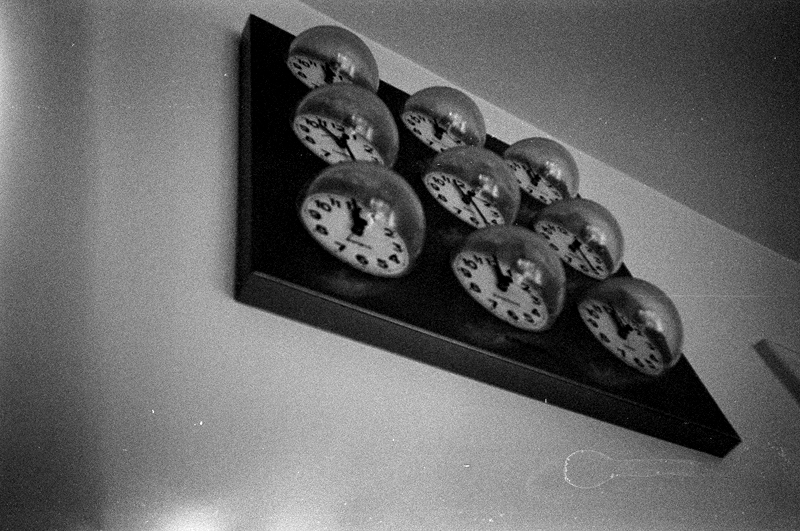A striking black-and-white photograph captures an intriguing installation viewed from a low angle. The focal point is a large black square mounted on the wall. On this square, nine identical small clocks are uniformly arranged in a 3x3 grid, each encased in a clear glass bubble. The clock faces are white, featuring black numerals and black hour and minute hands. Despite their uniform appearance, each clock displays a slightly different time, creating a subtle yet mesmerizing discrepancy. The wall and ceiling lie flush with each other, appearing to be the same monochrome hue, adding to the minimalist aesthetic of the scene. To the right, the edge of a door frame is just visible, hinting at the room's architectural layout.